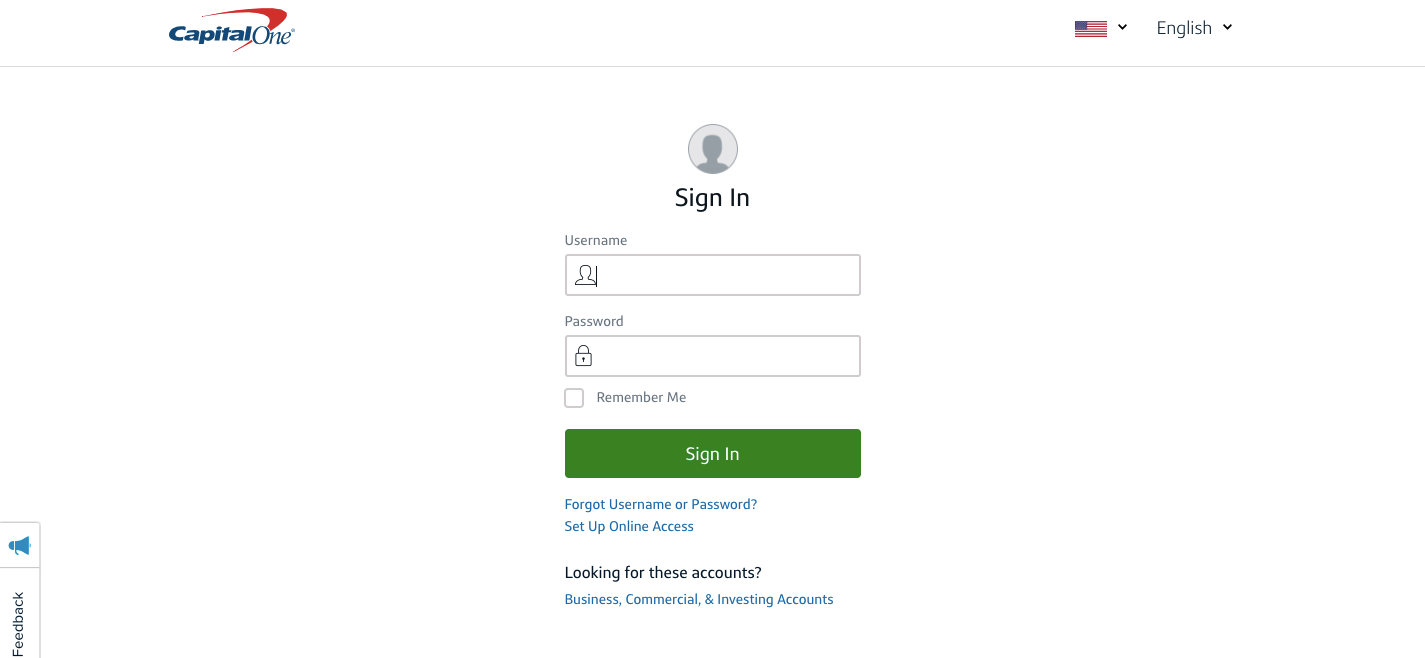The image depicts the Capital One sign-in page, characterized by a clean and structured layout with a predominantly white background. 

In the top left corner, the "Capital One" logo is prominently displayed with a distinctive red swoop, the text itself rendered in a bold blue font. Adjacent to this, on the top right corner, an American flag icon is accompanied by a dropdown menu for language selection, defaulted to English.

A horizontal gray line divides the header from the main content of the page. Centrally positioned is an avatar icon, showcasing a gray outline of a person's head and shoulders against a lighter gray circular background. Directly beneath this icon are the words "Sign-In" in black text.

The user input fields follow in sequence, beginning with a rectangular "Username" field marked by a subtle gray outline and a small person icon inside. The subsequent "Password" field mirrors this design, identified by a lock icon.

Beneath these fields, there is an unchecked "Remember Me" checkbox outlined in gray. Below this, a prominent green "Sign-In" button with white text invites users to proceed with their login.

Additional support links are provided below the button in blue text, including "Forgot Username or Password" and "Set Up Online Access." Further down, the text "Looking for these accounts?" appears in black, followed by blue hyperlinks for "Business," "Commercial," and "Investing Accounts."

The entire interface maintains a minimalist theme, emphasizing functionality and ease of use against a clean white backdrop.